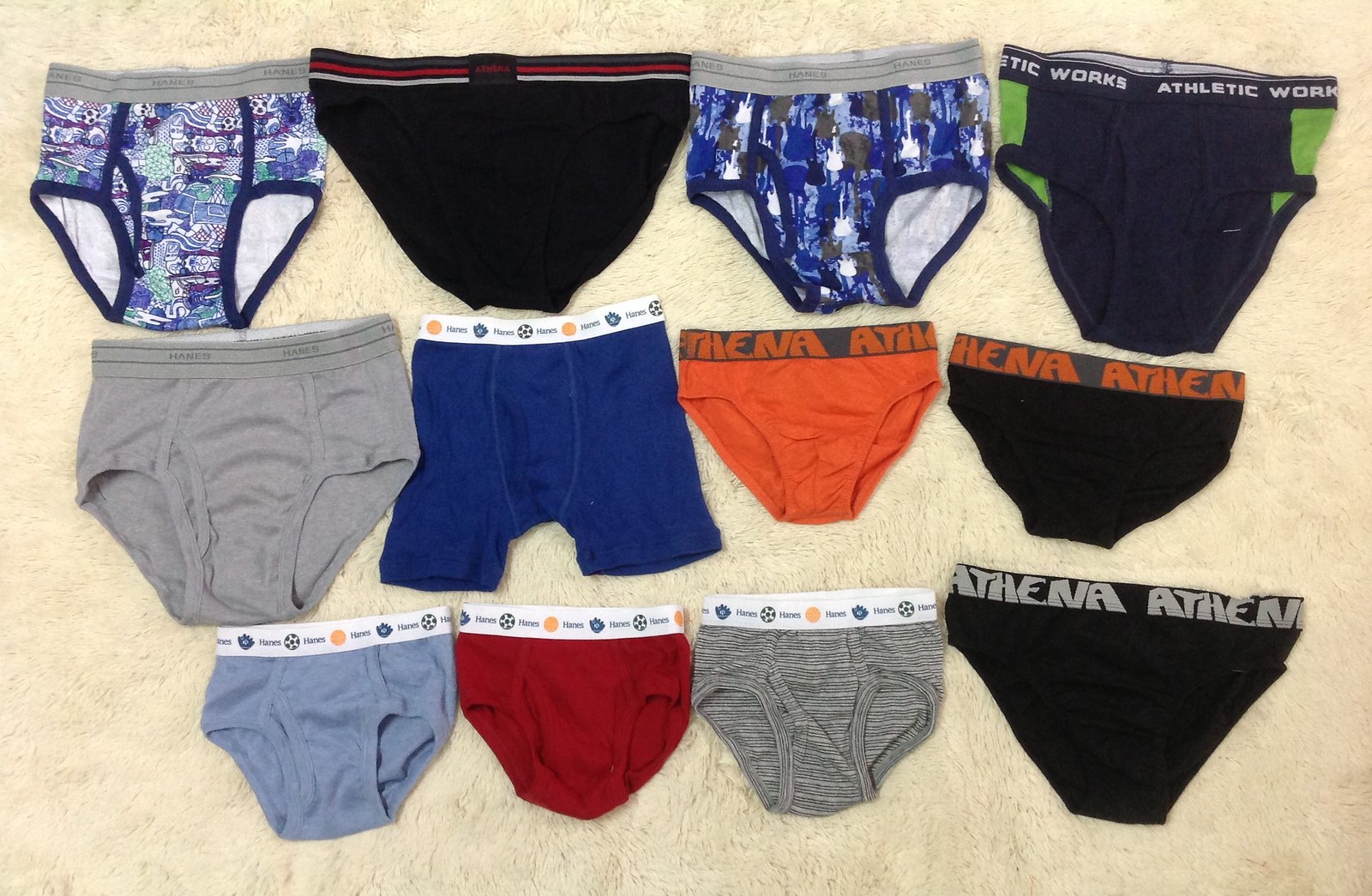The image depicts a neatly arranged collection of 12 pairs of young men’s underwear, laid out in three rows of four on an almost whitish tan carpet. These undergarments include a variety of brief and boxer brief styles, each in different colors and patterns. Starting from the top left, there is a pair with blue designs, followed by a plain black pair, then blue with little guitar motifs, and a black and green pair. The second row features an all-gray pair, a blue pair with a white border, a pair in solid orange, and black with an orange waistband. The bottom row includes a pair in blue, one in red, one gray and black, and another predominantly gray with black trim. The underwear showcase a mix of plain colors and intricate designs, including digital blue camo and comic book motifs.